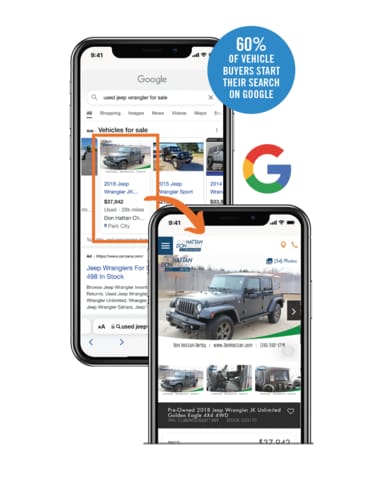The image showcases two cell phones, both with dark gray frames, with their screens prominently displayed. The phone in the background is on the Google search page, depicting search results that feature a vehicle highlighted by a vertically oriented orange rectangle. An orange arrow extends from this highlighted frame, directing attention to the screen of the second phone in the foreground. On this second phone's screen is an enlarged image of the highlighted vehicle, which is identified as a gray Jeep. Directly below the main image of the Jeep are three smaller pictures. In the top right corner of the overall image, a large blue circle contains white text that reads, "60% of vehicle buyers start their search on Google."